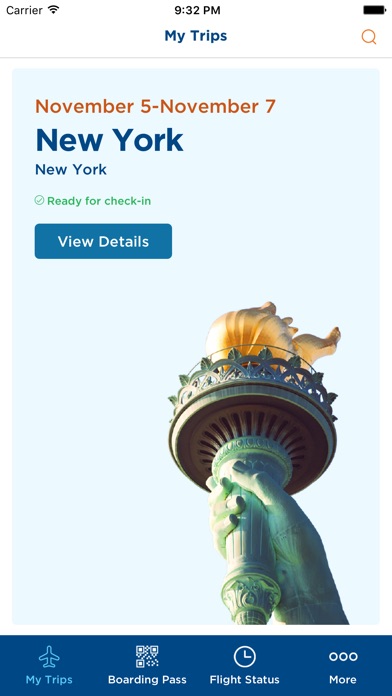The image is a screenshot from the MyTrips app displayed on a smartphone. At the top of the screen, the title "MyTrips" is prominently displayed. Below, there is a blue box in the lower right corner featuring the iconic hand of the Statue of Liberty holding a gleaming torch with a yellow flame.

At the top of the screen, clear orange text indicates the travel dates: "November 5 to November 7." Beneath this, the destination "New York" is displayed in bold blue print, with a smaller blue print repeating the destination "New York." Further below, green text proudly states "Ready for Check-In," accompanied by a check mark encased within a circle.

A blue rectangle labeled "View Details" with white print stands out against the blue background near the bottom of the image. Directly below this, in the blue box containing the Statue of Liberty's hand, several options are laid out in white print: "MyTrips," "Boarding Pass," "Flight Status," and "More," the latter being marked by three vertical dots. The "MyTrips" option is highlighted in blue, indicating it is currently selected.